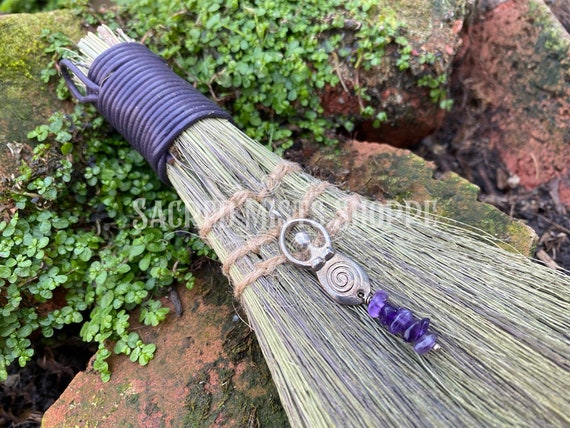An enchanting image of a handmade, decorative broom captured outside on a moss-covered stone porch. The broom, crafted from various grasses tightly bound with purple wire at the top, lacks a long handle, making it perfect for hanging rather than sweeping. The wire, done in a navy blue and purple hue, secures the fanned-out grassy bristles adorned with multi-colored strands including white, purple, and yellow. Dangling from the top is a charming silver and navy blue charm attached to the stitched part, adding a whimsical touch. The stone surface beneath the broom is alive with moss, small green plants, and hints of algae, creating a rich, natural backdrop. Across the image, the phrase "Sacred Mist Shop" is prominently displayed in white letters, enhancing the mystical ambiance of the scene.